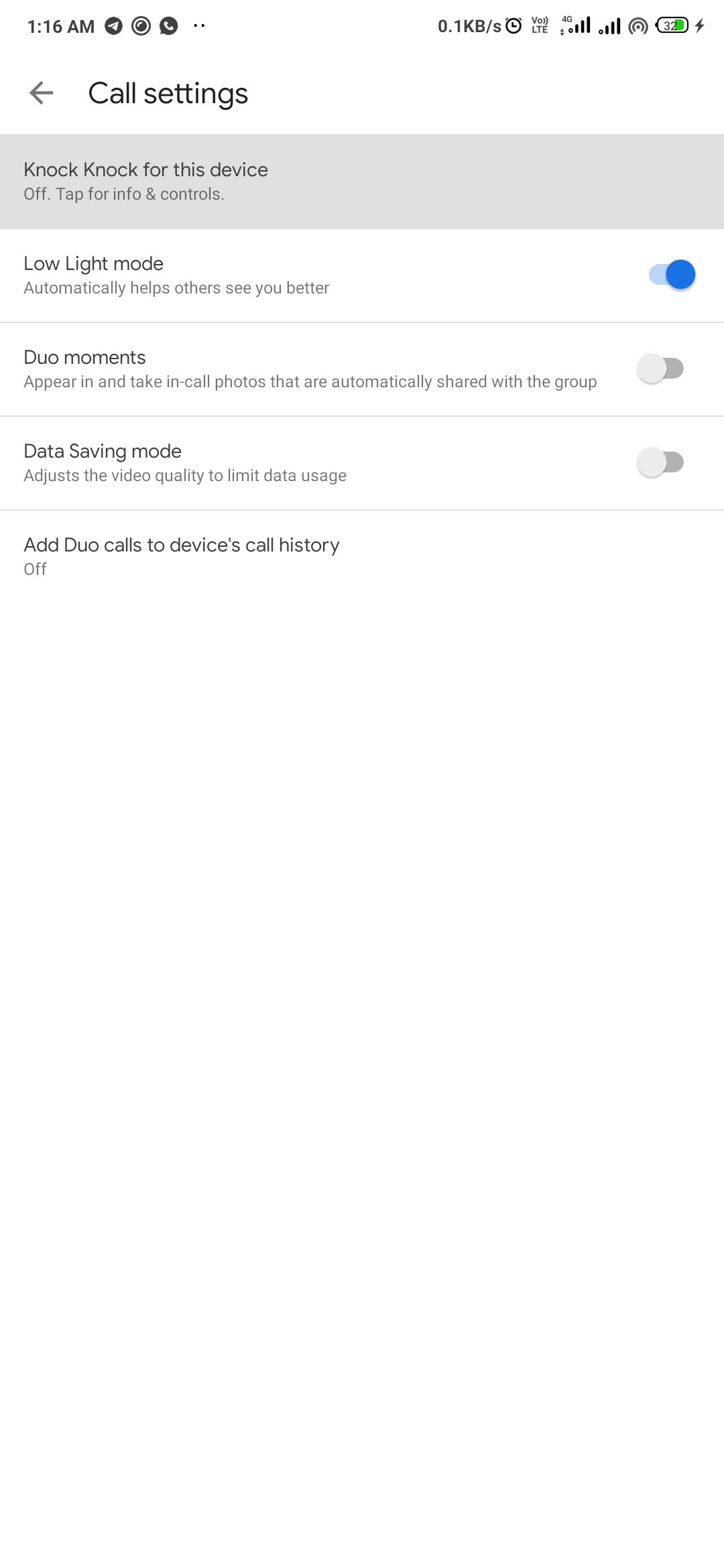**Caption:**

This image captures the screen of a cell phone on the "Call Settings" menu. 

In the top right-hand corner, various status icons are visible: 
- A charging icon
- A partially green battery icon
- An RSS feed-like icon
- A full bar cell signal icon
- A 4G cell service icon with full bars
- An LTE logo
- A clock indicating data transfer at 1.1 kilobytes per second

In the top left-hand corner, the time is displayed as 1:16 a.m., accompanied by:
- An arrow icon
- A camera lens-like icon
- A telephone icon inside a circle

Beneath this, a header titled "Call Settings" is present with a back arrow, indicating navigable options.

Below the header, several toggles and options are listed:
1. "Knock Knock for this device" is set to off, with a prompt to tap for more information and control.
2. "Low Light Mode" is enabled (shown by a blue switch), which helps others see you better during calls.
3. "Duo Moments," which allows in-call photos to be shared automatically, is switched off (gray switch).
4. "Data Saving Mode," which adjusts video quality to limit data usage, is also switched off (gray switch).
5. "Add Duo Calls to Device's Call History" is set to off as well.

Each option includes a concise description, and the overall screen layout is clean and functional, providing users with a straightforward interface for managing call settings.